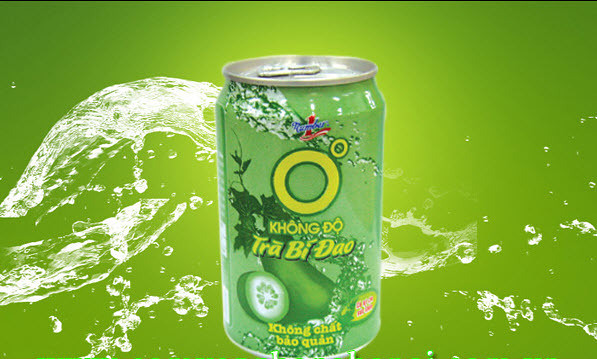A vibrant color photograph in landscape orientation features a bright green pop-top can prominently in the center. The can is topped with a chrome lid and has the pop-tab clearly visible. Central to the can's design is a bold yellow "O," accompanied by a smaller yellow "O" positioned at about the one o'clock mark. Elegantly presented at the bottom of the can is an illustration depicting a green vegetable, likely a cucumber, with a fresh slice of cucumber adjacent to it. The can is adorned with text in a language other than English, adding an exotic flair. The backdrop of this image is a lively lime green enhanced by a splash of water, emphasizing the refreshing nature of the beverage.